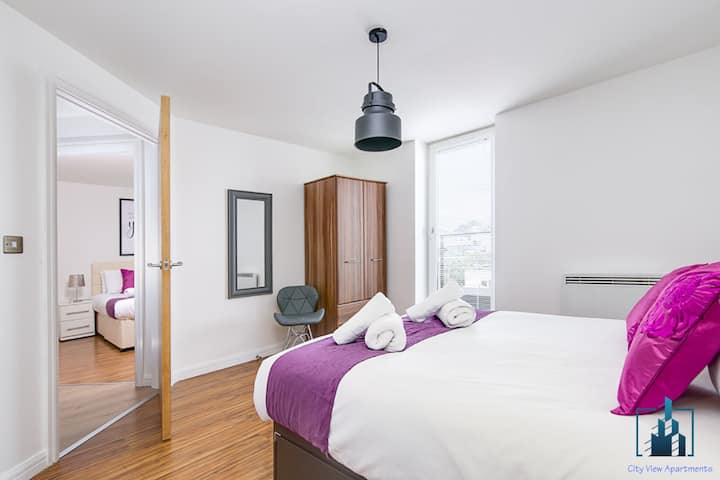This image showcases a photorealistic representation of a bedroom in City View Apartments, as indicated by the logo watermark in the bottom right corner. The apartment features a modern and minimalistic design with a color scheme of white, fuchsia, and gray accents. The bed, which dominates the room, is adorned with fuchsia pillows and a matching drape at the end, while the comforter is entirely white, complemented by four white towels. 

A medium-sized gray chair is positioned next to a dresser wardrobe that has a rectangular mirror on the far wall. This wardrobe with two doors provides ample storage space for clothes. The window, equipped with blinds, allows natural light to fill the room. 

The bedroom door on the left side is ajar, revealing a glimpse of another similarly styled room with analogous décor. A distinctive gray ceiling lamp hangs over the bed, adding to the modern aesthetic. The wooden flooring enhances the minimalist charm of the apartment. This thoughtfully designed space, part of a one or possibly two-bedroom layout, serves as an enticing advertisement for prospective renters.